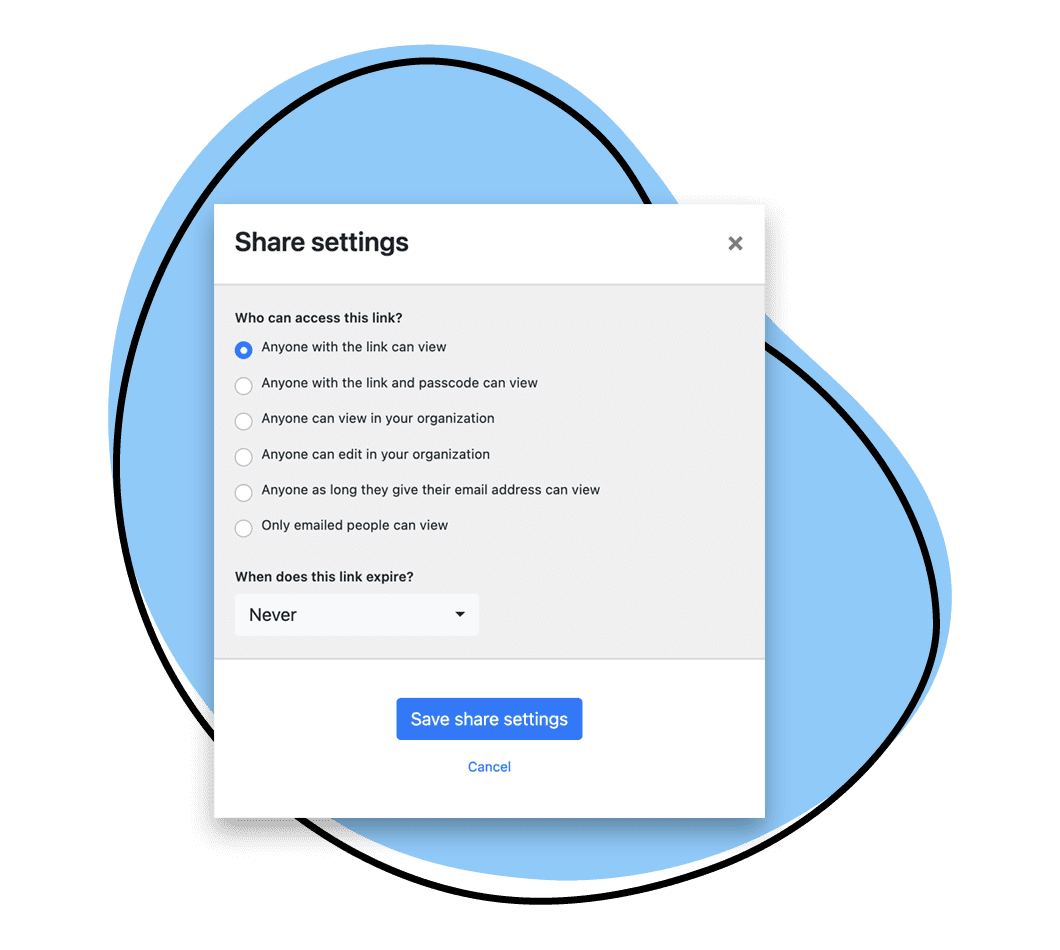The image features a user interface window of an application, set against an artistic background. The backdrop is designed with a playful, bean-shaped outline in black, partially filled with a light blue color that appears to be scribbled in, giving it a casual, hand-drawn vibe.

The user interface window itself is neatly divided into three sections. The top section, the smallest of the three, contains bold black text that reads "Share Settings," accompanied by a close (X) icon on the right end.

The middle section addresses link access options with bold black text, smaller than the top text, stating "Who can access this link?" This section presents several radio button options:
1. The first option is selected by default and reads, "Anyone with this link can view."
2. "Anyone with this link and passcode can view."
3. "Anyone in your organization can view."
4. "Anyone in your organization can edit."
5. "Anyone, as long as they provide their email address, can view."
6. "Only specific email addresses can view."

Following these options, the text "When does this link expire?" appears in bold, accompanied by a dropdown menu showing "Never," which is the selected expiry setting.

The bottom section contains two interactive elements: a blue button labeled "Save Share Settings" and directly beneath it, a blue cancel link that reads "Cancel."

This detailed interface layout efficiently communicates the sharing settings and permissions associated with a link, allowing users to easily configure and save their preferences.